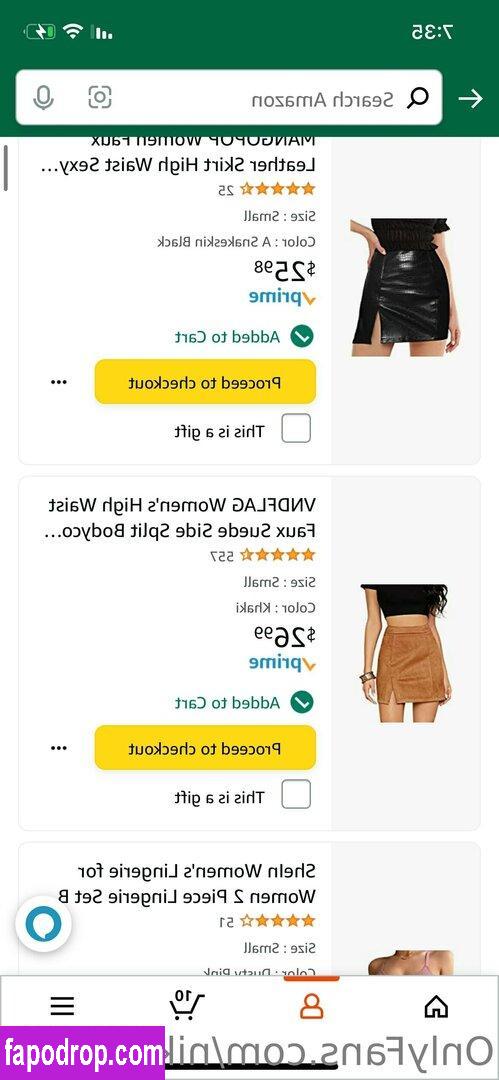This image is an inverted screenshot taken on a cell phone, depicting a page from the Amazon app, possibly Amazon Prime. The page has been flipped horizontally, causing everything that should appear on the left to be on the right and vice versa. Featured prominently on the right side of the shot are two women's skirts: one black and one beige, each with their individual prices listed beside them. A conspicuous yellow checkout button is also visible next to the skirts.

At the top right of the image, the time, displayed in reverse, reads 7:35. Directly below the time is a search bar containing foreign text, indicating that the entire webpage is in a foreign language. The bottom section of the screenshot shows a portion of the website's description, also reversed, yet still legible as "Only Fans." Additionally, the bottom left corner includes the partially visible text "fa-po-drop.com," suggesting another website link.

The overall visual context clearly indicates that this inverted screenshot captures a moment from browsing women's clothing on the Amazon app, viewed in an unfamiliar language, and incorporates notable elements like pricing, the checkout option, and peripheral web details.